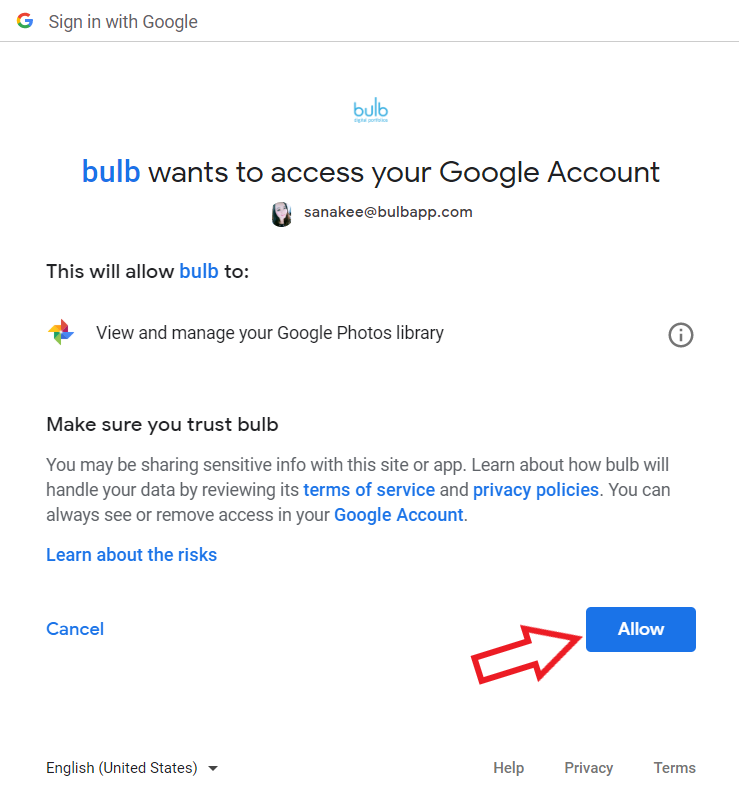The image demonstrates a Google sign-in authorization page for an application named "Bulb." 

- **Top-left corner:** The Google "G" logo appears followed by the text "Sign in with Google" in gray.
- **Central area:** There is a horizontal gray line separating the top section from the content below. Beneath it, the text "Bulb" appears in blue multiple times. Subsequently, in black text, it says "wants to access your Google Account."
- **User information:** A circular icon displays a woman's face alongside the email address "s-a-n-a-k-e-e@bulbapp.com."
- **Permissions:** Bulb requests the following permissions listed in blue: "View and manage your Google Photos library."
- **Security reminder:** A gray-outlined circle with an "i" inside is visible next to a cautionary message: "Make sure you trust Bulb. You may be sharing sensitive information with this site or app. Learn about how Bulb will handle your data by reviewing its Terms of Service and Privacy Policy." The words "Terms of Service" and "Privacy Policy" are clickable links in blue.
- **Account management:** Text in gray explains that users can always see or remove access to their Google accounts.
- **Additional links:** "Learn about the risks" is written in blue.
- **Action buttons:** Below, there are two main action buttons - "Cancel" on the left and a prominent blue "Allow" button on the right with a red outline pointing to it.
- **Footer section:** The bottom of the screen includes language settings displaying "English (United States)" with a downward arrow for a dropdown menu, and links for "Help," "Privacy," and "Terms."